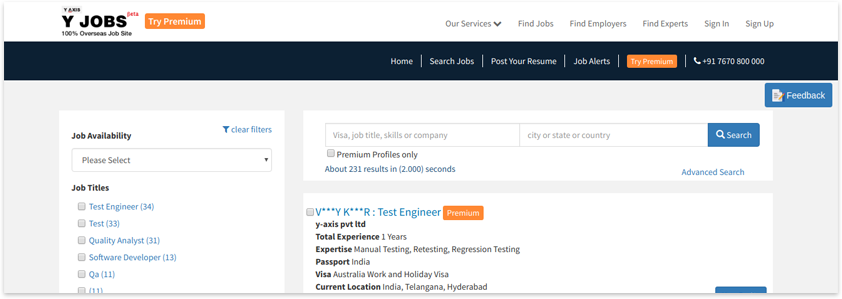This image is a screenshot from the YJobs website, currently in its beta phase. At the center bottom, it advertises itself as a "100% Overseas Job Site" and highlights the option to "Try Premium" with text in orange. At the top of the page, a series of tabs provide navigation options including "Our Services," a drop-down menu, and links for "Find Jobs," "Find Employers," "Find Experts," "Sign In," and "Sign Up."

Further down, the site shifts to a black background with a horizontal navigation bar that offers options such as "Home," "Search Jobs," "Post Your Resume," "Job Alerts," and another "Try Premium" button in an orange box with white letters. The top right corner displays a contact phone number: 917-670-800000.

On the left side, there's a section labeled "Job Availability," flanked by a "Clear Filters" option on the right. A drop-down box labeled "Please Select" allows users to filter job titles, such as "Test Engineer," "Test Quality Analyst," "Software Developer," with additional titles like "QA" not fully visible due to the image's cutoff.

Towards the center and right, additional filters offer search fields for "Visa," "Job Titles," "Skills or Company," and "City or State." A "Search" button and a "Premium Profiles Only" option are also present, noting "231 results in 2 seconds." Over to the right, an "Advanced Search" option is available beneath.

The central area highlights a job listing for "Test Engineer" labeled "Premium," under "YS Access Pvt Ltd," detailing a total experience of 1 year and skills in "Manual Testing," "Retesting," and "Regression Testing." The applicant's passport is noted as from India, and their visa status is listed as having an "Australia Work and Holiday Visa." The current location of the job seeker is in India, with other locations listed such as Tel Ghana and HyperDAC. A "Feedback" button is situated closer to the top right, just under the phone number.